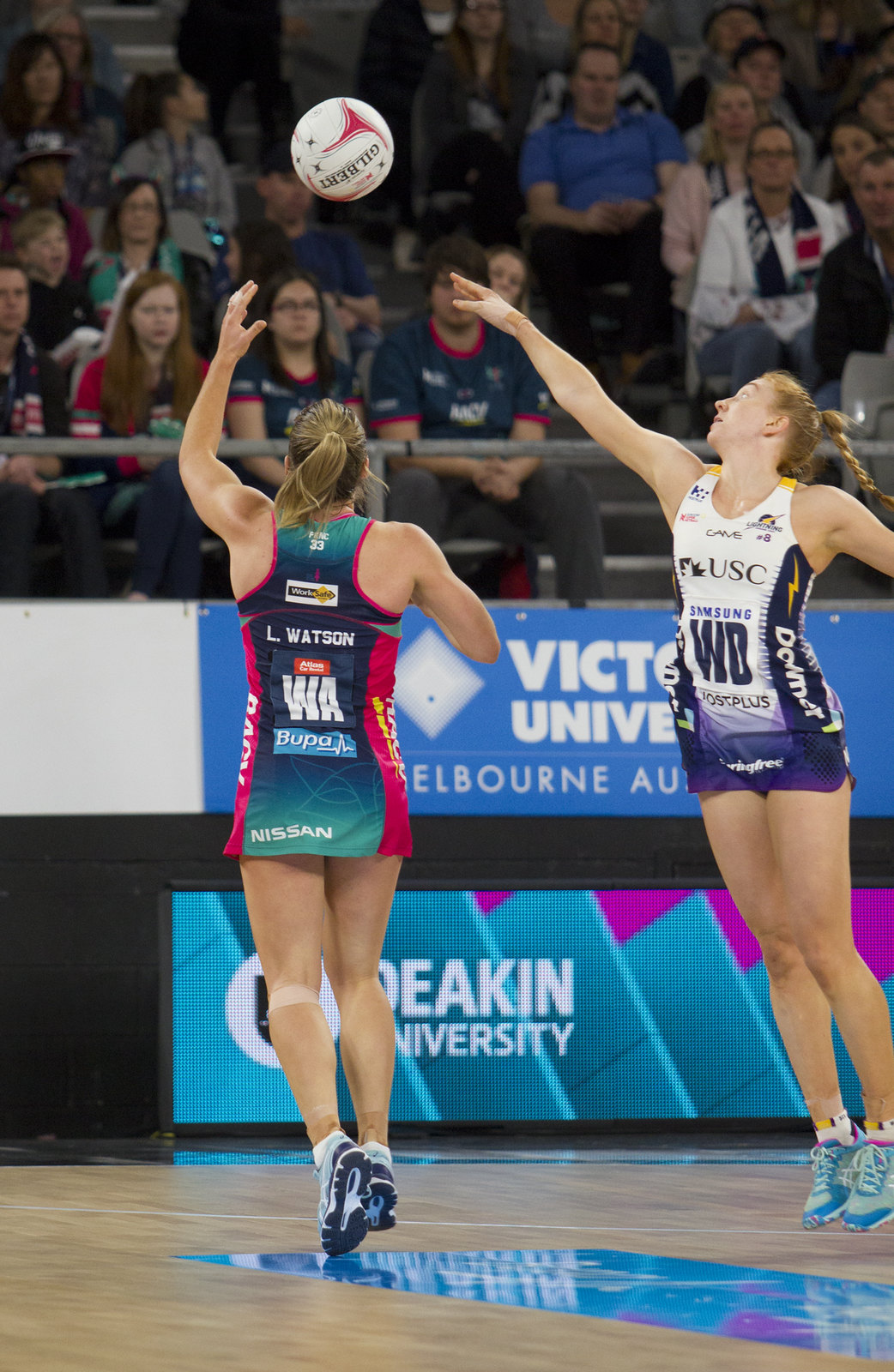This detailed image captures a thrilling moment of a women's volleyball game in an indoor stadium. The primary focus is on two female athletes poised mid-air, their eyes fixed on a white volleyball adorned with red designs, black stars, and some lettering, suspended near the top of the frame. The athlete on the left, her back to the camera, has blonde hair pulled back in a ponytail and wears a turquoise green and red uniform with the name "L. Watson, Washington, W.A." and the sponsor "Nissan" emblazoned on it. Her competitor on the right, donning a white and purple uniform with "USC, Samsung, W.D." written on it, is slightly closer to the ball.

They are positioned on a shiny wooden court with distinct blue rectangular markings. High above, gray railings and horizontal banners can be seen, and beyond them, the stadium's bleacher-style seating is filled with spectators who line either side of a central stairway aisle. Advertisements on the stadium front include VICT, UNIVE, and Melbourne, AU, indicating a university setting. Both athletes are wearing tank top-style uniforms and tennis shoes, showcasing their athletic readiness as they compete in this intense match.